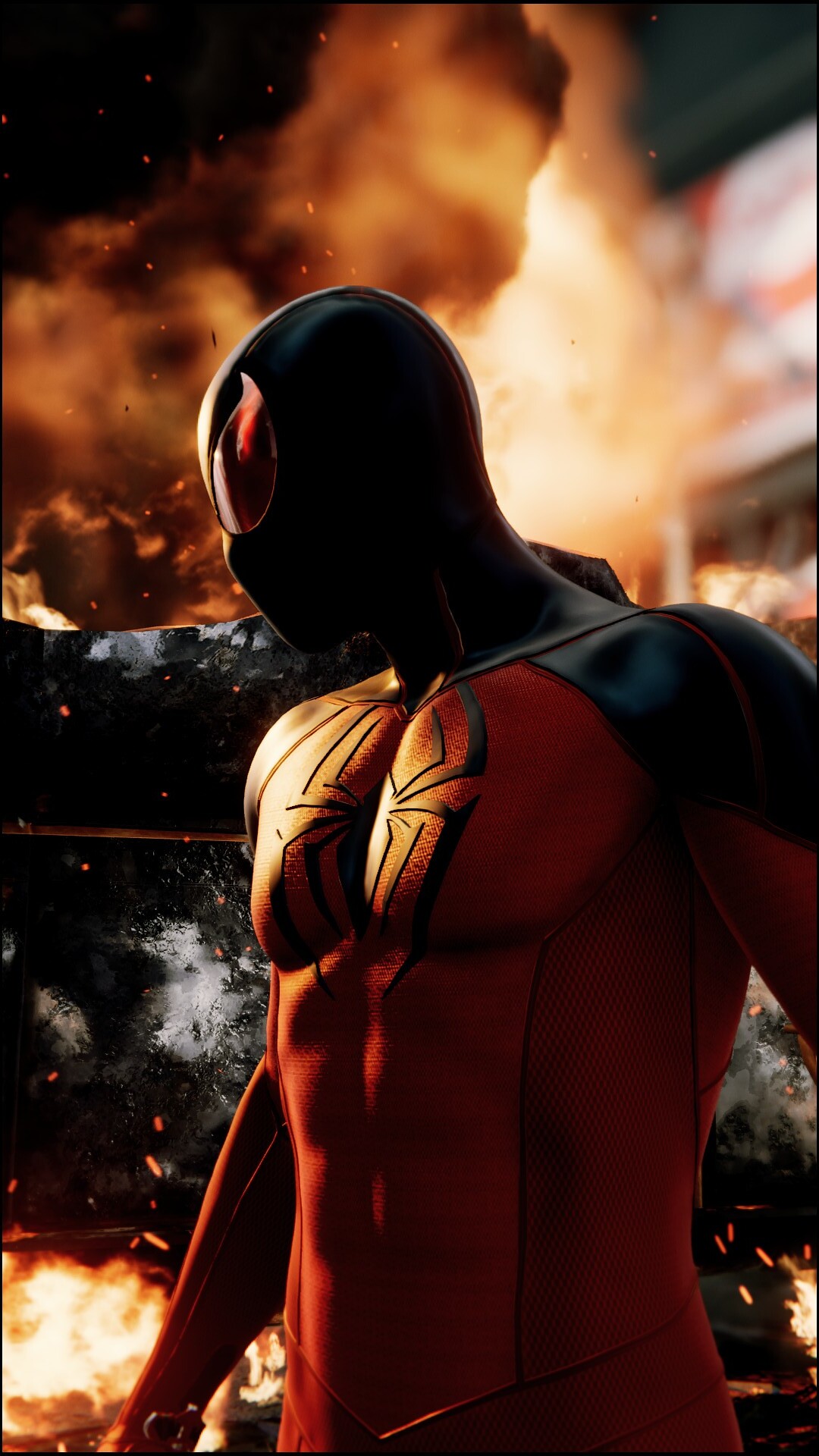This is a highly detailed, color photo of Spider-Man that appears to be animated or computer-generated with photorealistic quality. Spider-Man, who is featured from the head down to his waist, is gazing to the left. He is dressed in his iconic red suit with black shoulders and hood, highlighted by a black spider emblem on his chest. His reflective, red eye covers mirror the fiery chaos behind him. The background is a dramatic display of dark clouds, swirling black and gray smoke, vibrant orange flames, and intense explosions with glowing embers floating through the air, casting an orange glow that illuminates Spider-Man from the left. The setting appears to include rubble, suggesting a scene of destruction. The scene encapsulates a moment of intense action and danger.